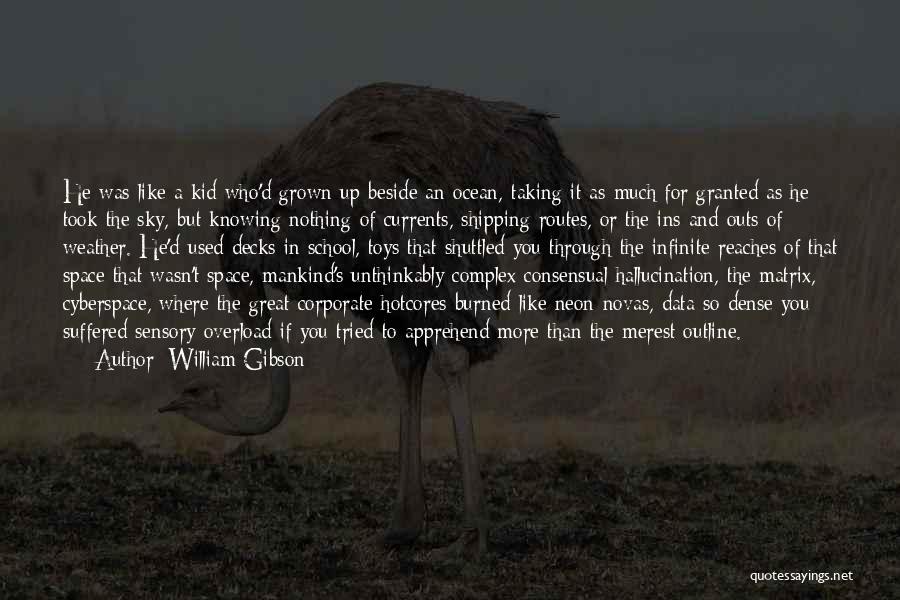The image from QuoteSaying.net features a quote by author William Gibson and depicts an intricate scene. The background is a dimmed, black-and-white image of an emu or ostrich standing in a field, facing left with its head bent towards the ground. The setting includes yellow grass and a dirt trail or road visible in the background, suggestive of a plain or savannah. The bird's fluffy brown feathers contrast with its bony legs, adding texture to the scene. Overlaying this serene landscape is the quote in white text, reading:

"He was like a kid who'd grown up beside an ocean, taking it as much for granted as he took the sky, but knowing nothing of currents, shipping routes, or the ins and outs of weather. He'd used decks in school, toys that shuttled you through the infinite reaches of that space that wasn't space. Mankind's unthinkably complex, consensual hallucination, the matrix, cyberspace where the great corporate hot cores burned like neon novas, data so dense you'd suffer sensory overload if you tried to apprehend more than the merest outline."

In the bottom right-hand corner of the image, the source "QuoteSayings.net" is noted, also in white text.